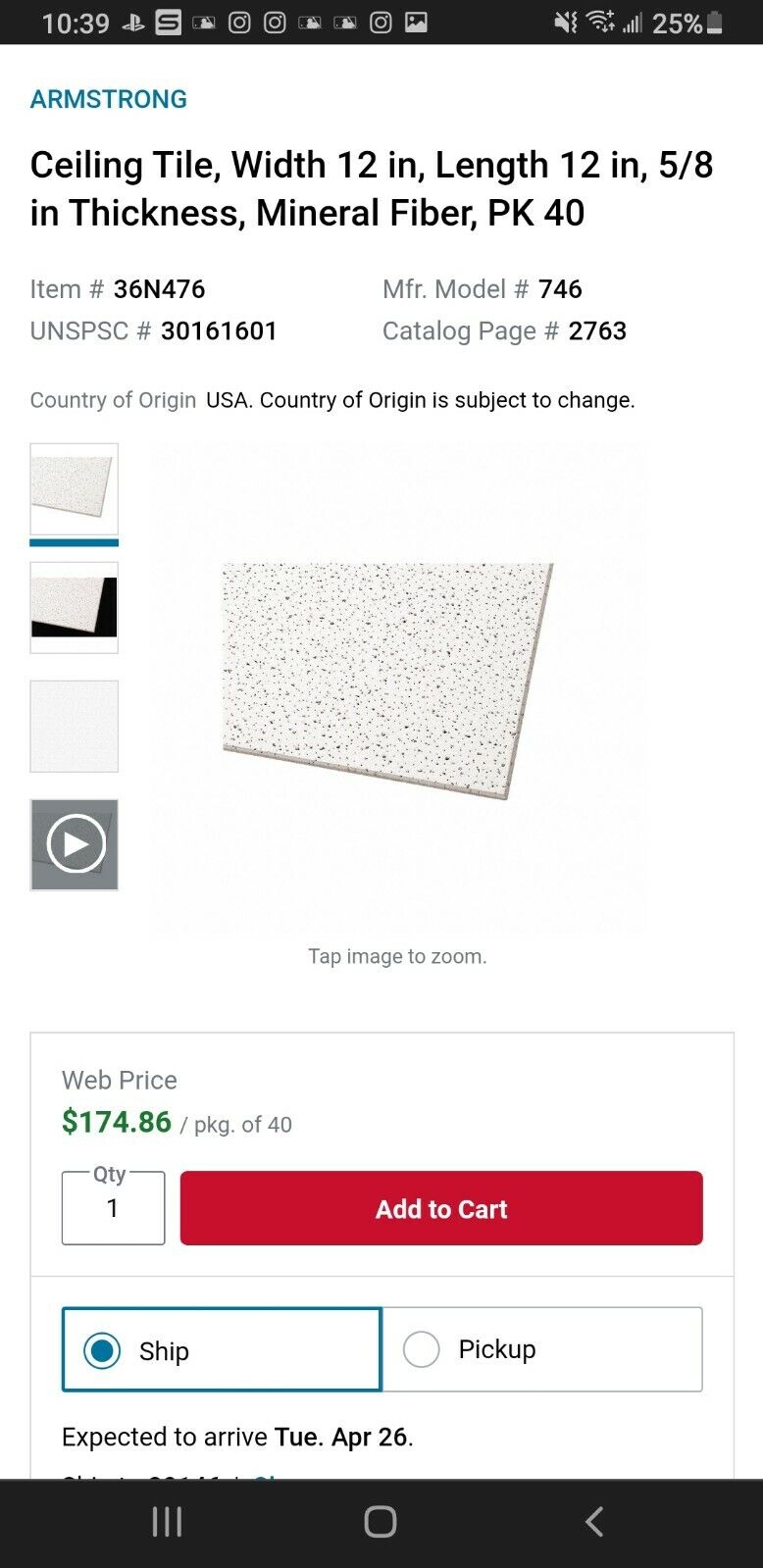**Product Listing for Armstrong Ceiling Tile**

This detailed product page showcases Armstrong ceiling tiles, providing comprehensive information and multiple ordering options. The primary product image is accompanied by several smaller images offering additional views, all formatted in a professional and clean layout with a plain white background to minimize distractions.

### Product Description:
- **Brand**: Armstrong
- **Product Type**: Ceiling Tile
- **Dimensions**: 
  - **Width**: 12 inches
  - **Length**: 12 inches
  - **Thickness**: 5/8 inches (5 and 8th)
  - **Material**: Mineral Fiber
- **Package Quantity**: 40 tiles
- **Item Number**: 36476
- **Manufacturer’s Model Number**: 746
- **UNSPSC Number**: 30161601
- **Catalog Page Number**: 2761

### Pricing:
- **Cost**: $174.86 for a package of 40 tiles
- **Pricing Section**: Uses bold red text to draw attention to the call to action.

### Ordering and Shipping:
- **Ordering Options**: Available for order on the product page.
- **Expected Arrival Date**: Displayed for user convenience.
- **Shipping Options**: Multiple choices including home delivery and store pickup.
- **Additional Features**: Offers "tap to zoom" functionality on the main product image for a detailed close-up view.

### Layout:
- **Background**: Plain white with minimal distractions.
- **Text Details**: Placed on the left side of the page while images are displayed on the right.
- **Professional Presentation**: Clean and easy-to-navigate design, ensuring a streamlined shopping experience.

Additional elements such as battery status and time are displayed at the top of the mobile device view, enhancing user convenience. This well-organized page ensures customers have all the necessary information to make an informed purchase.